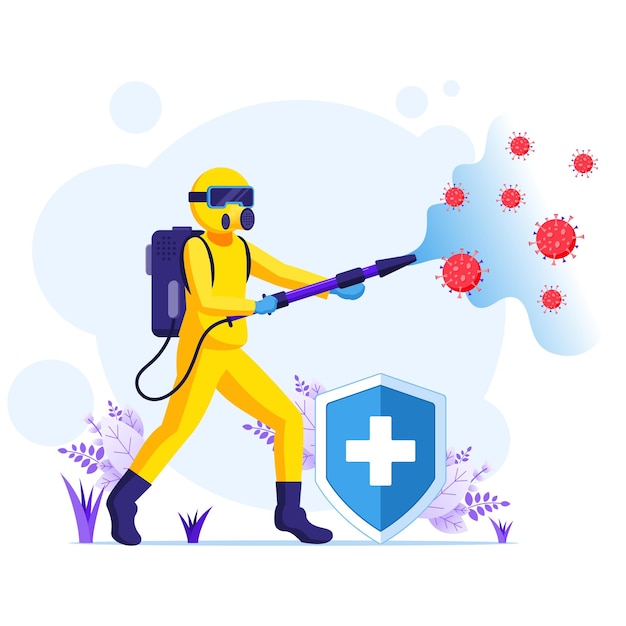In this simple two-dimensional cartoon illustration, a person is depicted in a full-bodied yellow hazmat suit, complete with a face mask, eye protection, gloves, and blue boots. The individual is fully equipped with a blue backpack that is connected by a purple hose to a wand they are using, which emits a mist containing red virus-like microbes, reminiscent of the coronavirus with its iconic spiked appearance. They seem to be combating the virus in a quarantined environment. 

A prominent blue shield with a white cross, suggesting a medical context, is positioned beside the person. The background is a light blue and white gradient, giving it a cloud-like appearance, while the ground and surrounding area feature sprouting and scattered purple plants, adding a splash of color to the otherwise minimalistic scene. The visual elements collectively create an impression of the character actively disinfecting or fumigating the area, possibly symbolizing efforts to fight off viral pathogens.